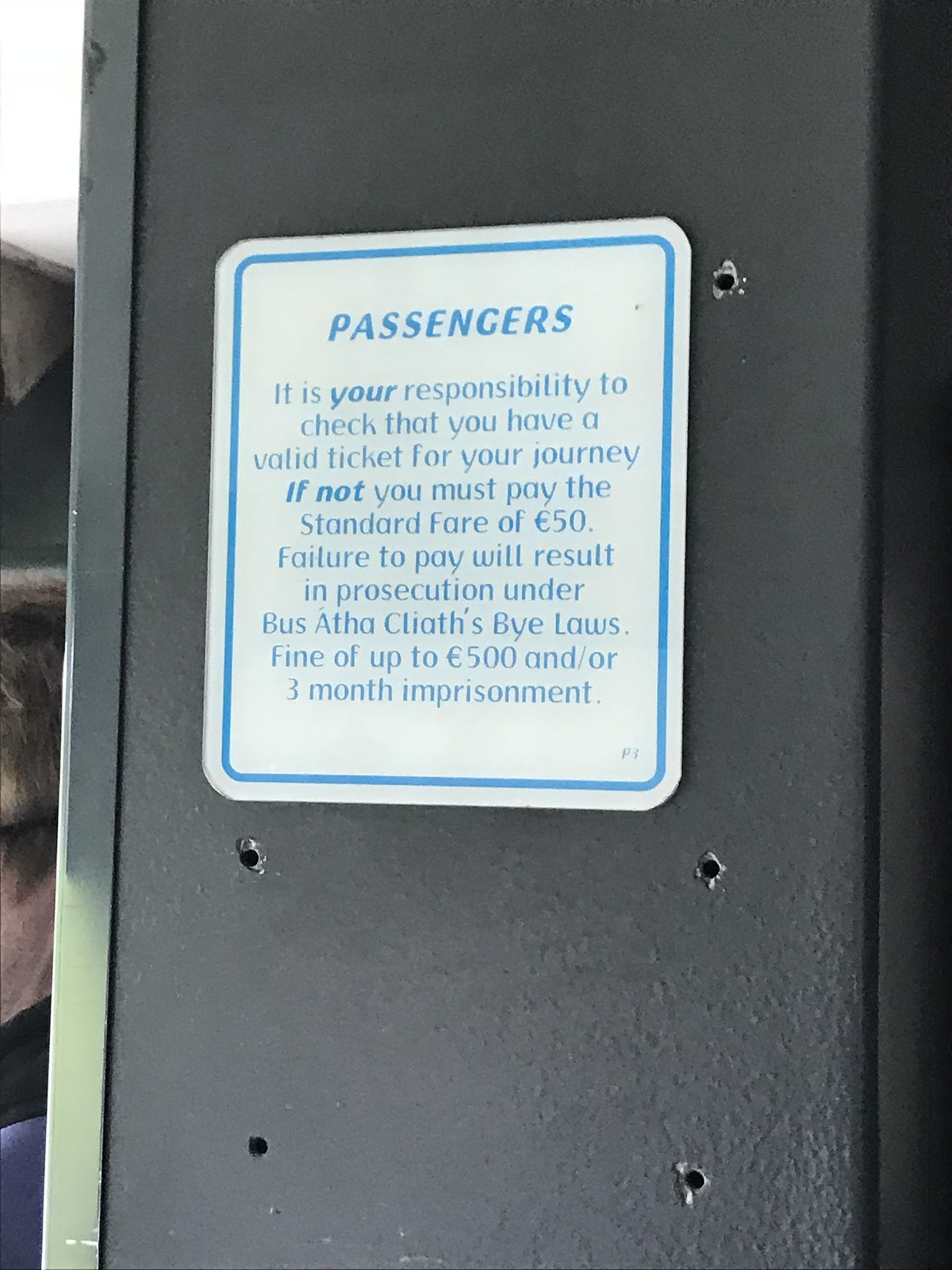This image captures a close-up of a rectangular sign, affixed to a grey metallic girder, likely within a public transportation setting such as a train or bus. The sign features a white background with a distinct blue border and blue text. It prominently displays the word "PASSENGERS" at the top in bold blue letters. Below this heading, the sign informs in smaller blue print: "It is your responsibility to check that you have a valid ticket for your journey. If not, you must pay the standard fare of €50. Failure to pay will result in prosecution under Bus-Atha-Cliahs Bylaws, a fine of up to €500, and/or three months imprisonment." The image also shows the sign mounted on a larger black structural beam with a light silver vertical border on the left side. The beam has pre-drilled holes that remain visible around the sign. A partially blurred face is subtly visible on the left edge of the image, adding a human element to the scene.